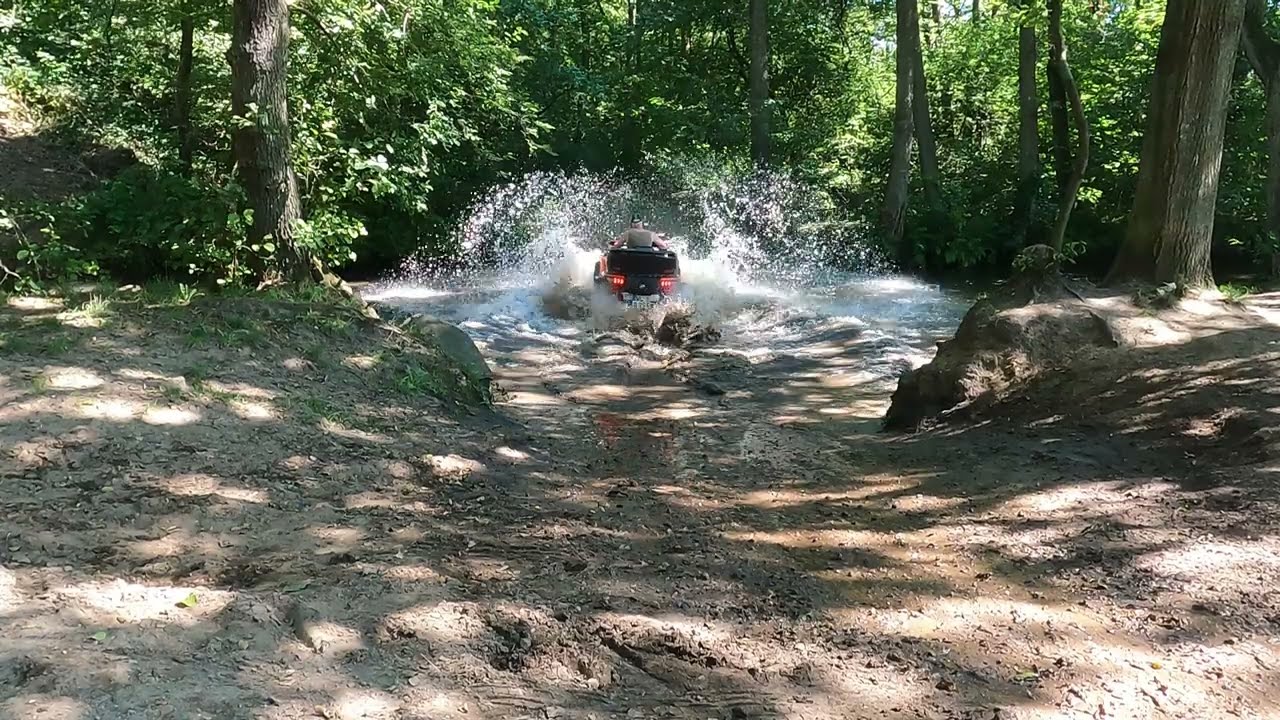A vibrant outdoor scene unfolds in this photograph taken during a sunny day in what appears to be summer. In the image, a man drives an all-terrain vehicle (ATV) through a shallow creek, with water splashing everywhere as he rides away from the camera. The ATV's taillights are lit up, and tire tracks reveal he has just traversed a muddy, dirt path. The watery area is flanked by ground that slopes slightly upward, bordered by numerous trees. These trees create a lush, green canopy that allows sunlight to stream through their leaves, casting dappled light across the scene. The path ahead appears to lead deeper into the dense, wooded area, which is teeming with greenery and vegetation.